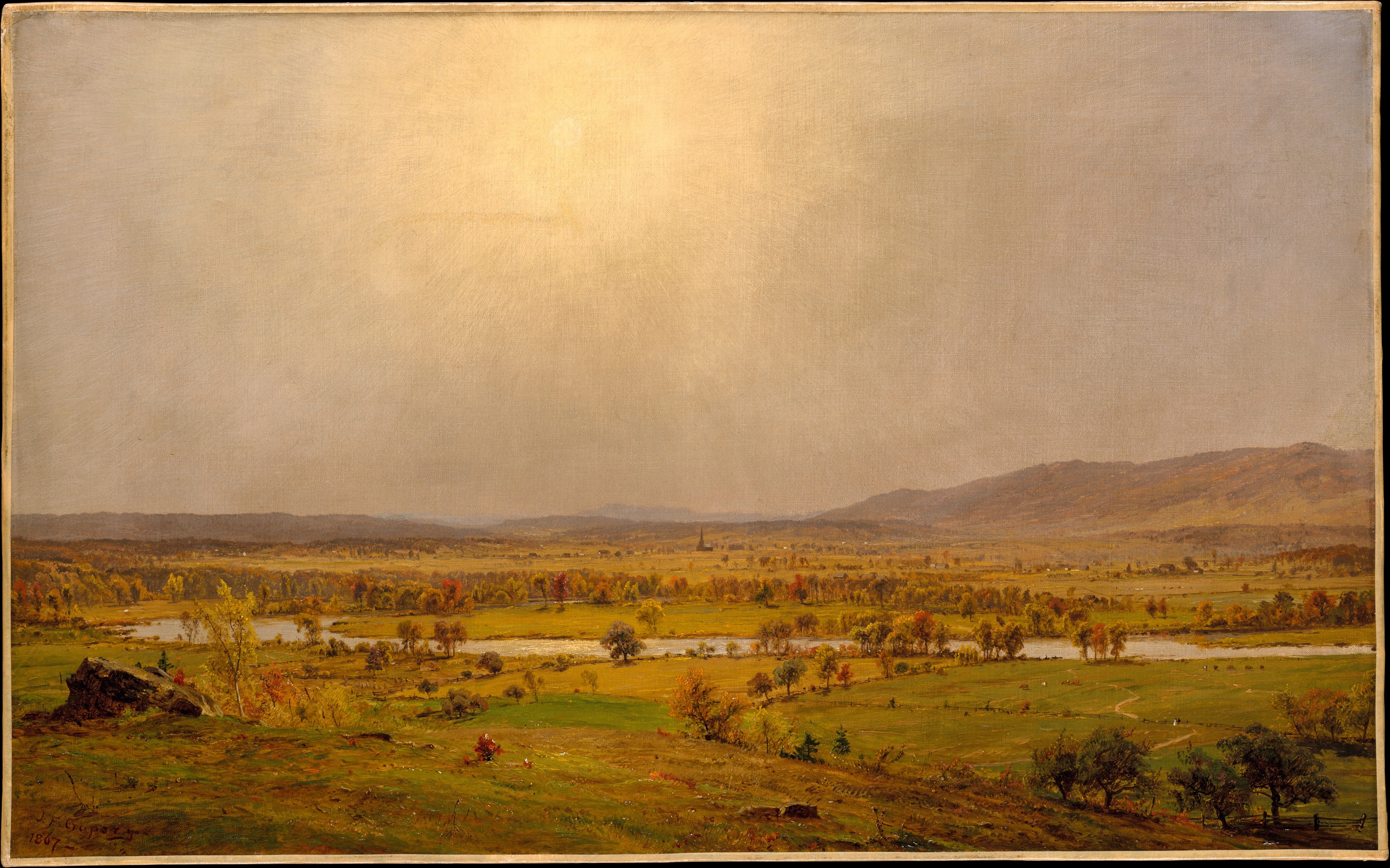The painting depicts a detailed and expansive country landscape, showcasing an autumnal scene with vibrant orange and yellow foliage. In the middleground, a serene river or pond extends from the left-hand side to the right, bordered by clusters of trees. The ground features a mix of yellow and green hues, peppered with rocks. The scene is framed by distant mountains on both the left and right sides. The sky presents a muted, overcast atmosphere with hints of pinkish-gray and blue, partially obscuring the sun which is positioned slightly to the left of the center. In the background, there appears to be a small church, barely noticeable unless closely examined. A farmhouse is situated on the lower left, contributing to the pastoral feel of the painting, while a path leading to the river can be observed on the right side. The artist's meticulous attention to detail suggests a scene that feels both expansive and intimate.